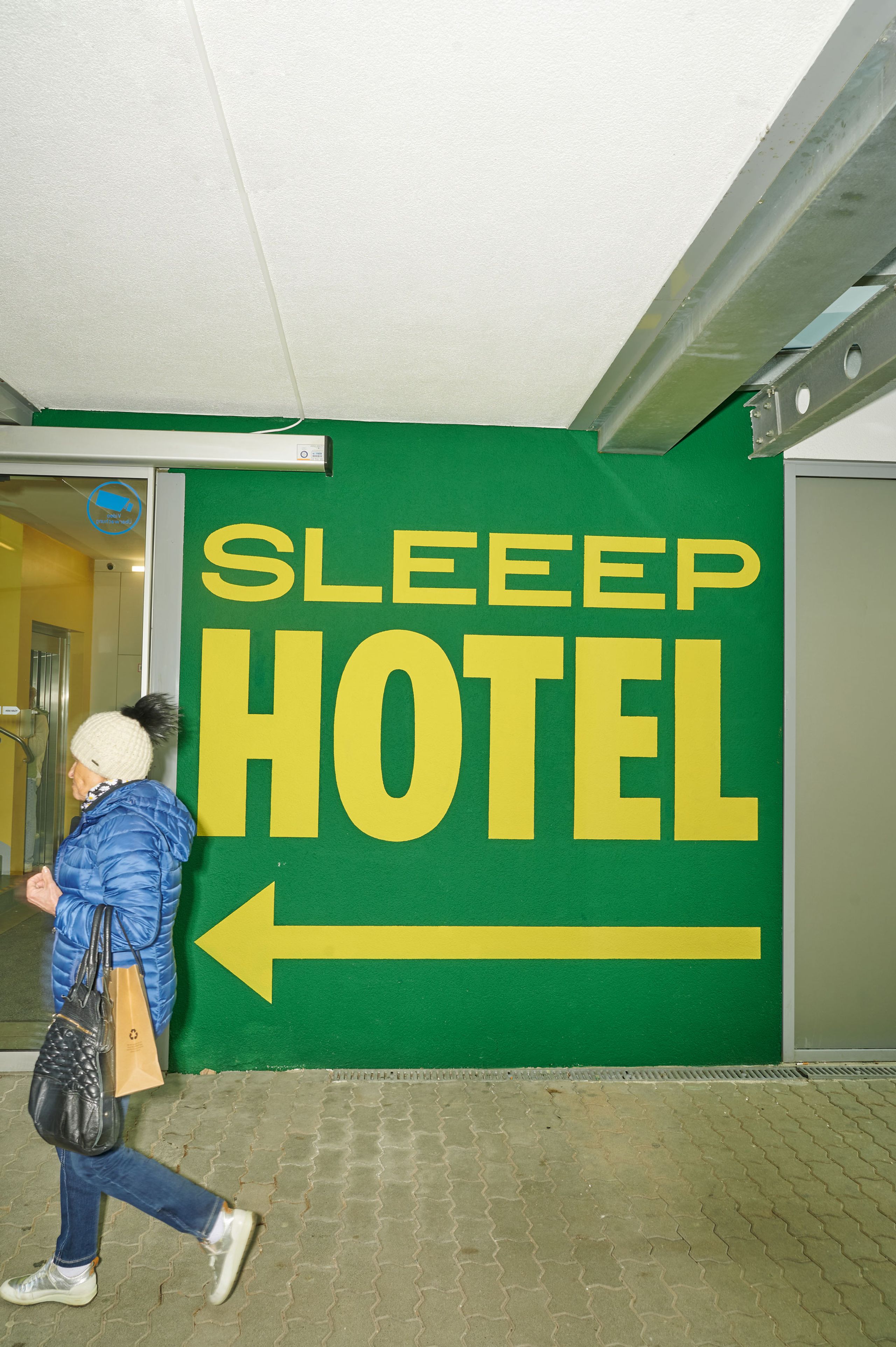In this detailed interior image, a woman is walking to the left side of a building's corridor. She wears a blue, puffy jacket, blue jeans, and white and silver shoes with a white sole. A black leather purse hangs from her shoulder, and she also carries a brown paper bag. A white hat with a black pom-pom tops her outfit. The floor beneath her is a concrete surface made of pavers, and the ceiling above is white with metal fixtures and beams.

Dominating the wall behind her is a large green banner with the word "SLEEP" spelled with three E's in large yellow letters, followed by "HOTEL" in matching yellow font. Below "HOTEL," a yellow arrow points to the left, indicating the direction to the hotel. To the right of the green banner is a grey wall, while on the left, there is a window with a blue icon resembling a security camera in the top right corner. The area has an overall appearance of a somewhat neglected indoor space, with dirty beige floors adding to the worn-out feel. Additionally, there are some glass doors adjacent to the green banner, contributing to the hallway's function as a passageway in the building.